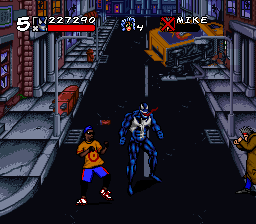The square image resembles a vibrant, cartoon-like scene from a video game. Dominating the center is a black road that runs vertically through what appears to be a bustling cityscape. On the right side of the road, the base of city buildings and a sidewalk are visible, suggesting a neighborhood street. Similarly, on the left side, another sidewalk flanked by city buildings is shown, with a prominent street lamp jutting out.

In the bottom section of the image stand two distinct figures on the road. The central figure is non-human, entirely blue, adorned in a silver vest, with a matching blue helmet or mask, and a conspicuous red tongue protruding from its mouth. To its left is a human figure with dark skin, dressed in blue shorts, an orange T-shirt, a blue cap, and sunglasses. This figure has arms extended as though preparing to punch.

Additionally, in the lower right corner of the image, there is another character of ambiguous identity, clad in a brown jacket. Only the profile and outstretched arms of this person or creature are visible, positioned as if ready to engage in combat, facing west.